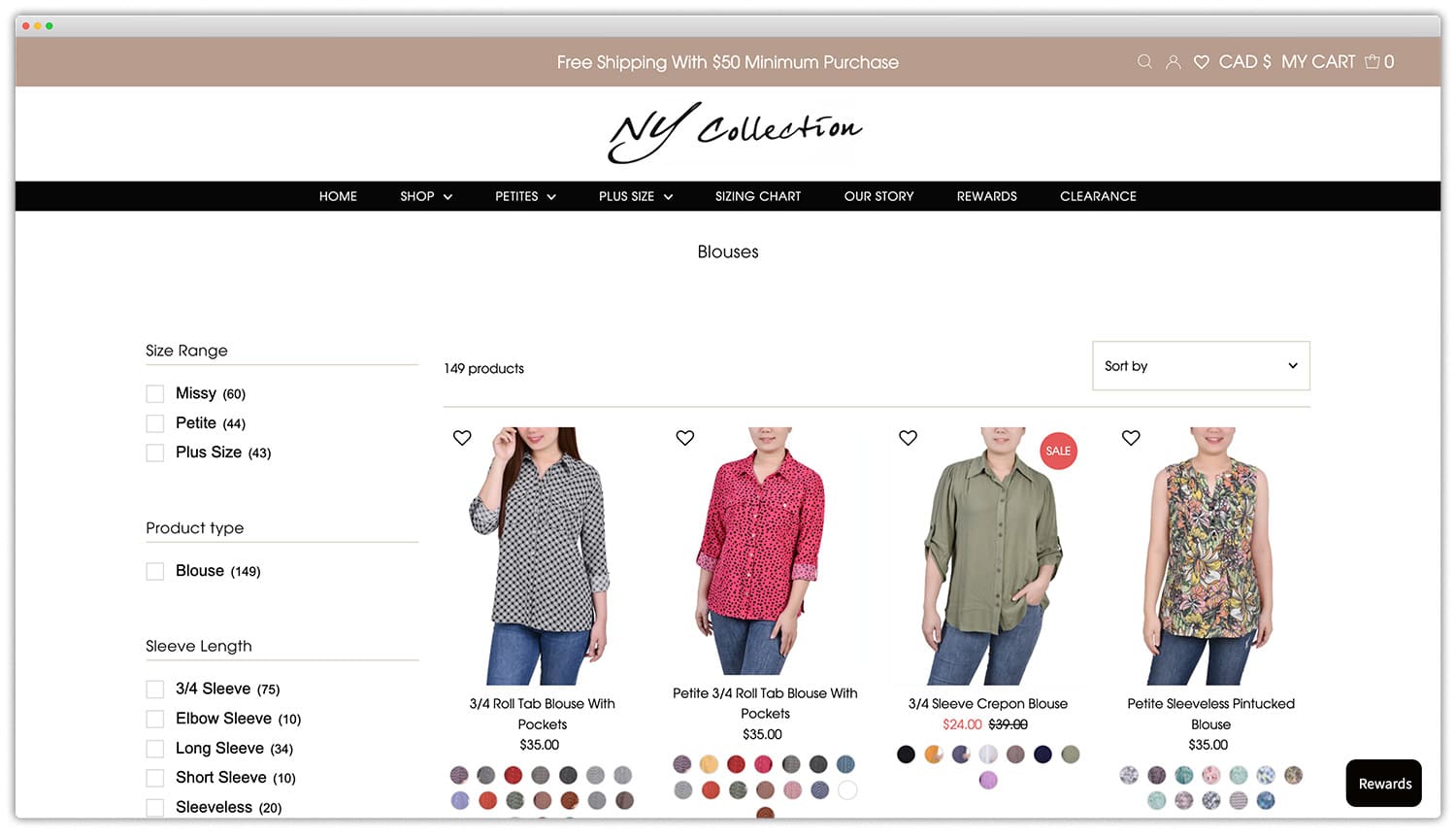Screenshot of the "New York Collection" fashion website, showcasing a diverse array of women's outfits. The collection includes a variety of shirts, such as polka dot and leopard print designs, with a selection of nearly 20 different patterns. The range of sizes is extensive, catering to Miss, Petite, and Plus Size categories. The product types include blouses with various sleeve lengths like 3/4th sleeves, elbow length, long sleeves, short sleeves, and sleeveless. The website allows users to sort products by sleeve length and other criteria. Navigation options are available for Home, Shop, Petite, Plus Size, Size and Chart, Our Story, Rewards, and Clearance. Additionally, the site features images of four women wearing different sizes to guide shoppers.